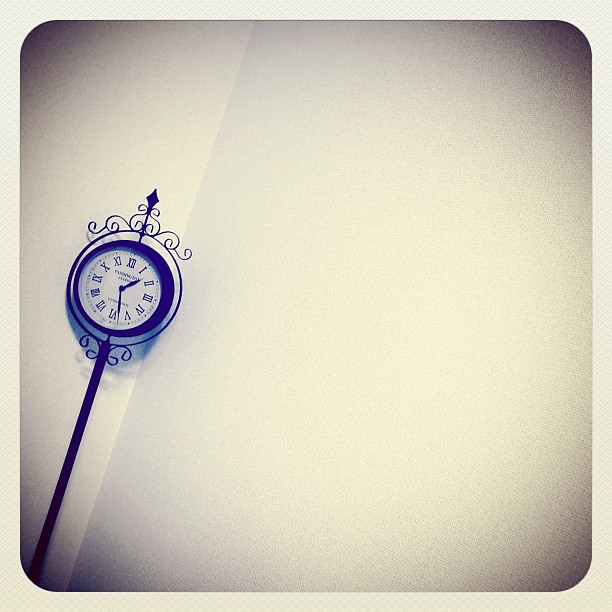In this intriguing photograph, a gray wall dominates the background, gradually fading to white on the left side. At the bottom left corner, a clock is perched atop a slender pole. This clock features ornate black edges at each corner, specifically at the bottom left, bottom right, top left, and top right. Adding a touch of elegance, the clock is crowned with a small, pointy triangle at the very top. The sides of the clock display gentle curves on both the left and right.

The clock face is meticulously detailed with numbers from 1 to 12 encircling it. Above and below the center of the face, there are texts that are not fully legible in this image. The hour hand is positioned between the 1 and 2, while the minute hand is situated between the 5 and a symbol resembling a 'B' or 'I'. To further enhance its intricate design, the clock face includes dash marks around its circumference. The interplay of light and shadows in the photo creates a sense of depth, subtly casting shadows behind the clock and adding dimension to its appearance.